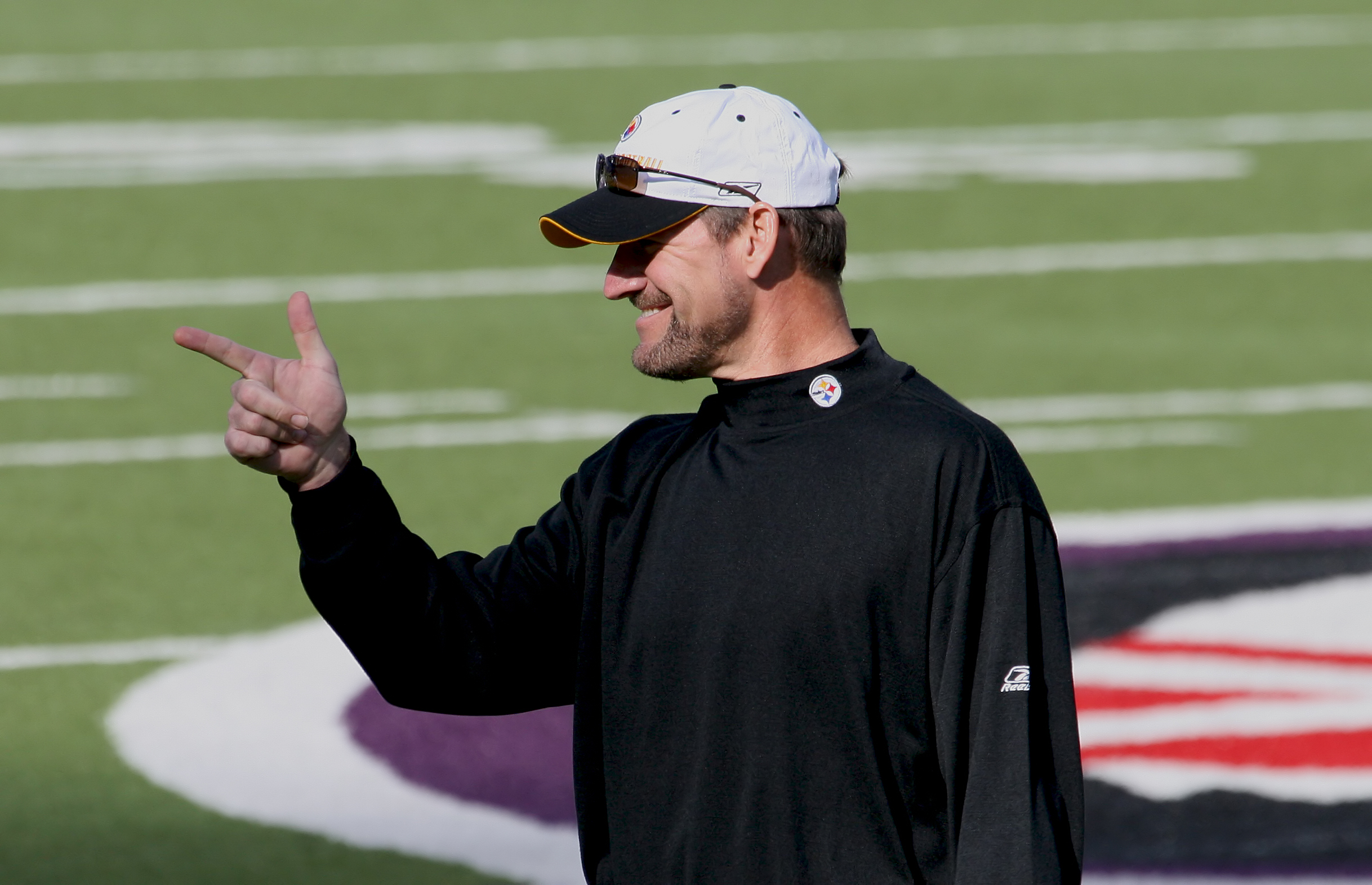A man, possibly an NFL player, stands on a sunlit football field, identifiable by the white lines and stripes across it. In the background, there is a large logo with colors including white, purple, black, red, and white, though its exact nature is unclear. The man is smiling broadly and pointing with his right hand, his thumb raised and index finger extended, towards someone or something in the distance. He is wearing a black Steelers Reebok sweatshirt, which has the Reebok logo on his left sleeve and the Steelers logo near the collar. He also sports a white cap with a black brim, with sunglasses perched on top, and has a beard, enhancing his casual yet engaged demeanor. The clear daylight suggests it is the middle of the day, adding to the vibrant atmosphere of the scene.